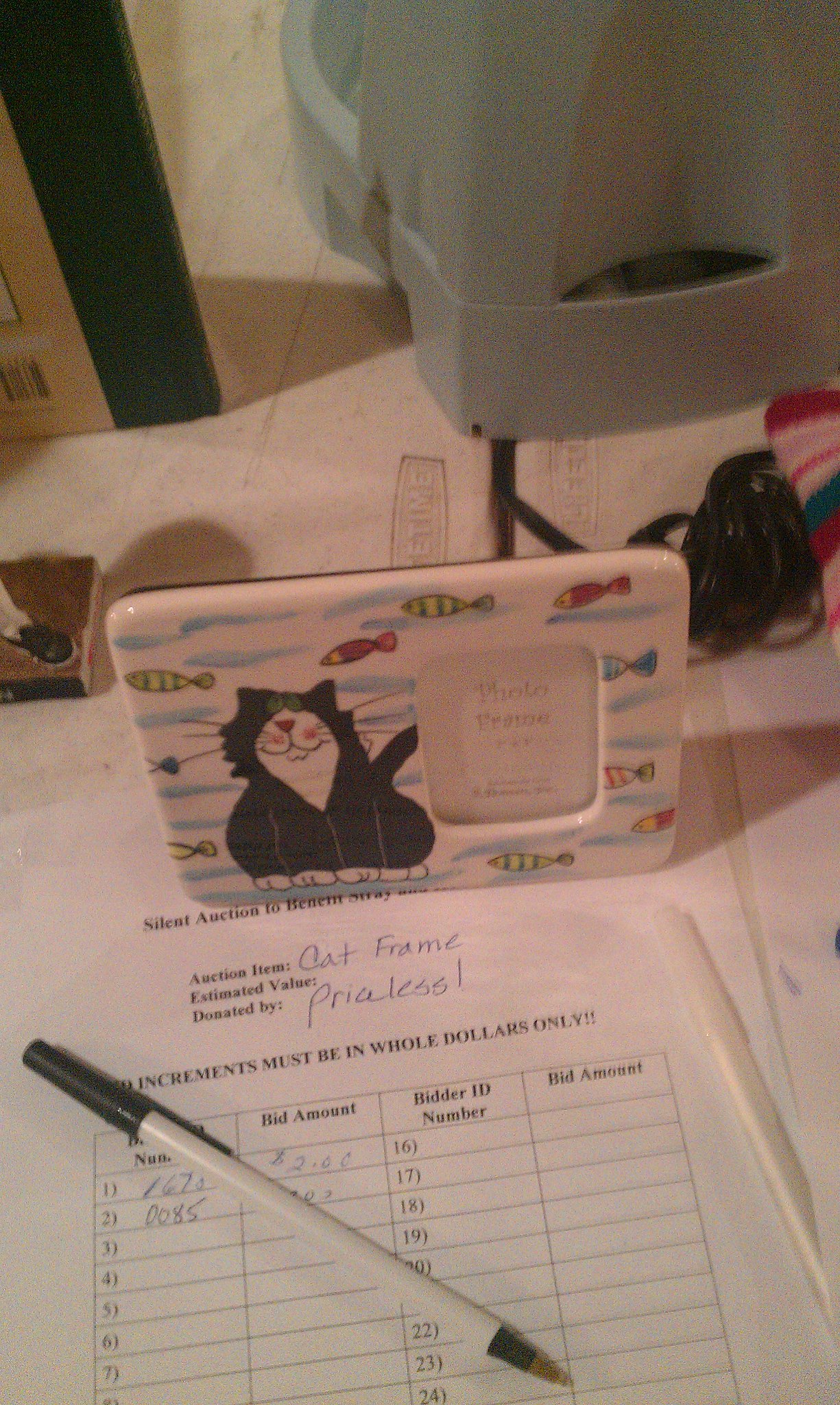The image is a rectangular photograph depicting a ceramic picture frame at what appears to be a silent auction. The frame features a black-and-white, comic-like illustration of a cat on the left side, surrounded by colorful fish—yellow, pink, blue, and green—set against a backdrop of swirling blue patterns that evoke a water scene. The right side of the frame has a small, square space, approximately two inches by two inches, intended for a photograph. Below the frame lies a printed bidding sheet labeled "cat frame priceless," with instructions that all increments must be in whole dollars. The sheet is structured with several numbered lines for participants to write their bidding number and bid amount. A black-and-white pen rests diagonally across the top of this sheet. Additional items, including a gray device, are visible on the light brown table surface behind the frame.